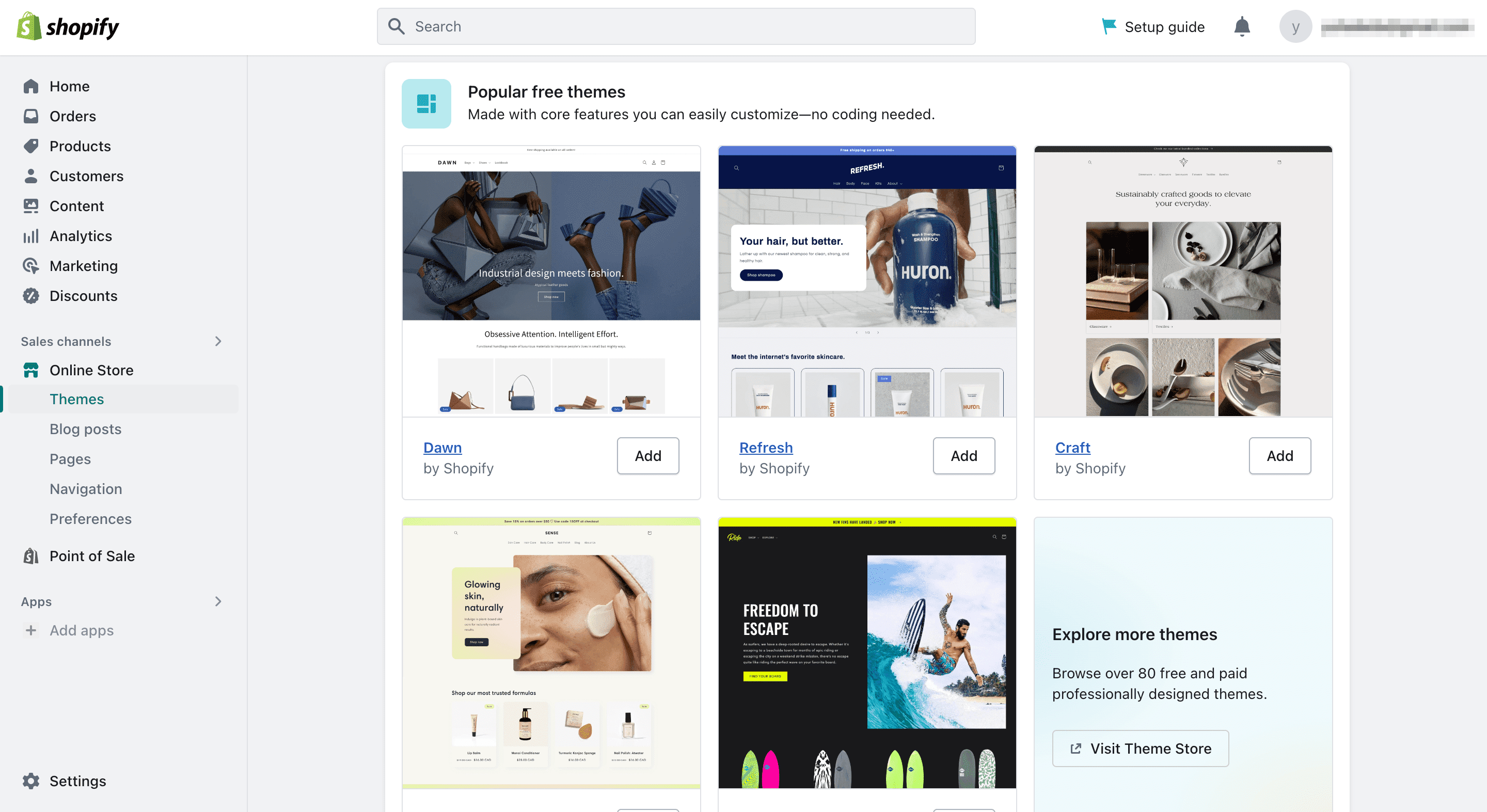This image showcases a Shopify web page user interface. The left pane features a comprehensive list of categories, including Home, Products, Customers, Content, Analytics, Marketing, Discounts, Sales Channels, Online Store, Themes, Blog Posts, Pages, Navigation, Preferences, Point of Sale (POS), Apps, Ad Apps, and Settings. A search bar is prominently positioned at the top. 

The main section highlights "Popular Free Themes" with a tagline emphasizing their core features, which are easily customizable without requiring any coding skills. Among the showcased themes are "Setup Guide," "Done by Shopify," "Refresh by Shopify," and "Crafts by Shopify." Additional text encourages users with the "Freedom to Escape" to explore more themes, with an invitation to browse over 80 free and paid professionally designed themes in the VC Theme Store.